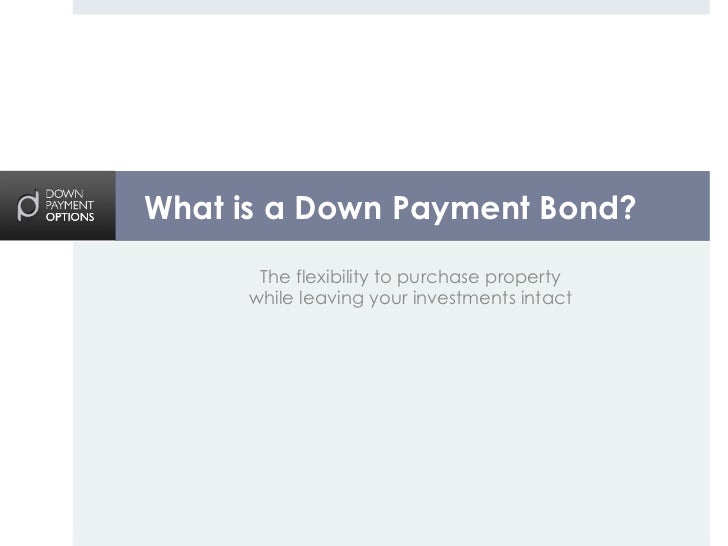The image showcases a slide from a presentation or website, featuring text organized to provide information about down payment bonds. A grey border frames the slide, with a corporate logo on the upper left corner, represented by the letters "DMP" stacked vertically. Next to the logo, a black box contains the text "Down Payment Options." Centered at the top, a white title on a light blue background poses the question, "What is a Down Payment Bond?" Directly below this, black text on a lime background answers, stating, "The flexibility to purchase property while leaving your investments intact." The overall layout includes a grey bar at the top and a predominantly white or light blue background, typical of an introductory presentation slide.